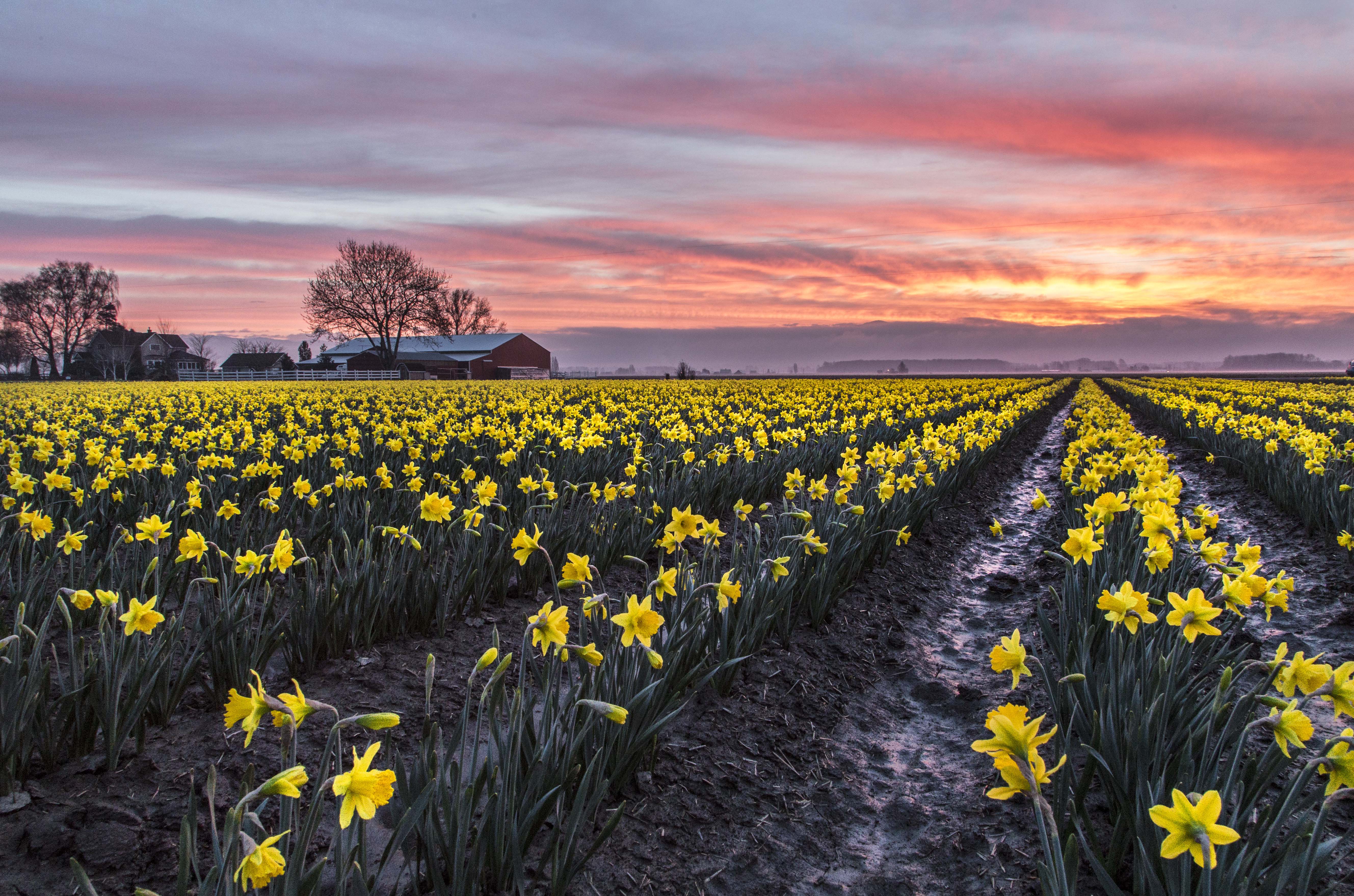The image depicts an expansive outdoor setting during either sunrise or sunset, characterized by vibrant hues of purple, pink, orange, and blue streaking across the sky. The foreground features long, evenly spaced rows of blooming yellow daffodils, their six-petaled flowers creating a harmonious and uniform field. Among the yellow flowers, green leafy plants add a touch of contrast. In the distant background to the left, a red barn, a house, and additional buildings are visible, surrounded by leafless trees and a white fence encircling the property. The entire scene is enveloped in the serene light of the setting or rising sun, highlighting the peacefulness of the rural landscape.